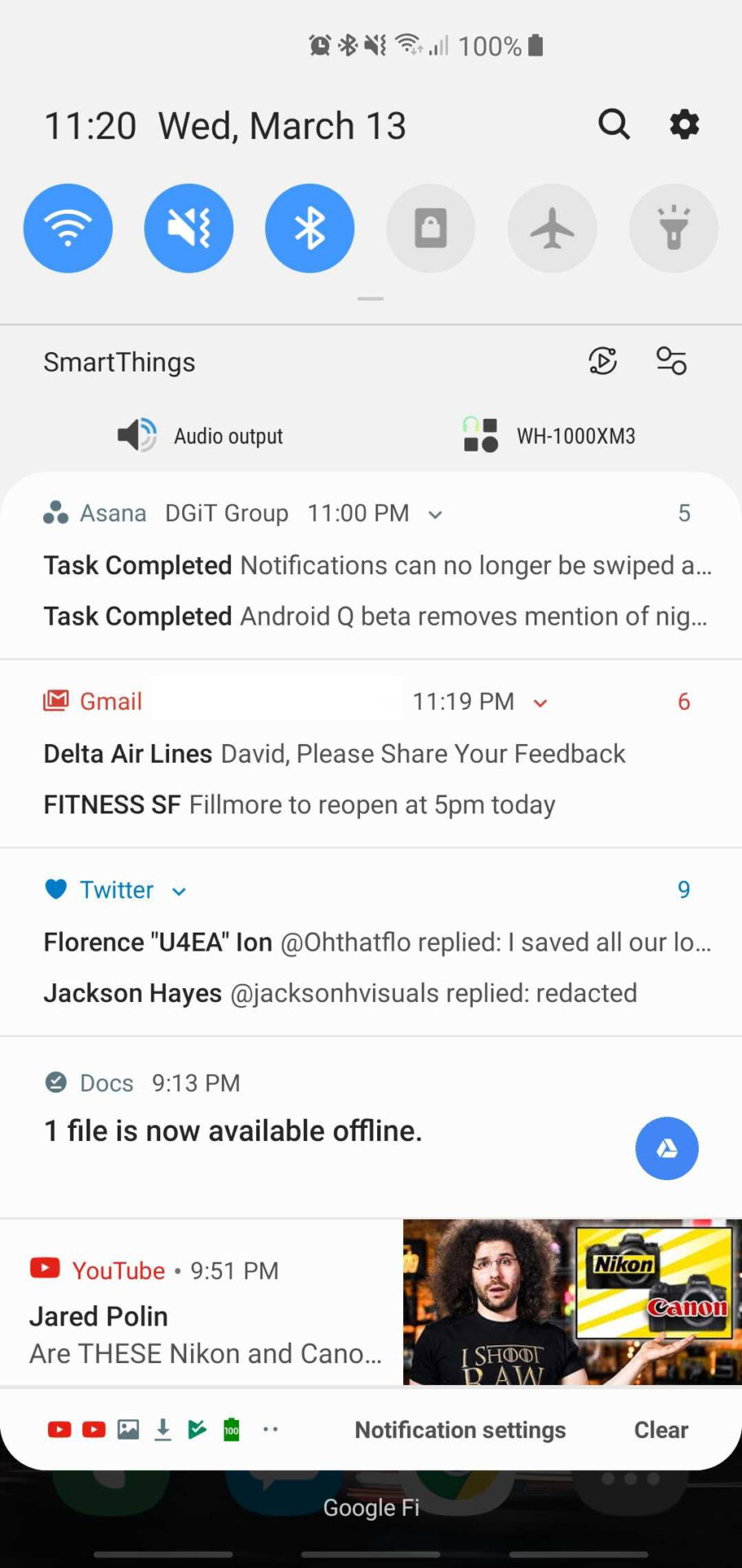This is an image of the Google Mail app interface on a smartphone. At the top of the screen, the time is displayed as 11:20 AM on Wednesday, March 13th. Adjacent to the time are several status icons, which include a clock icon, a Bluetooth icon, a no-ring icon, a Wi-Fi icon, and a work profile icon. The battery icon shows a 100% charge.

In the control icons below the date, several buttons are highlighted in blue, indicating they are active: the Wi-Fi button, the no-sound button, and the Bluetooth button. Other icons, such as the lock screen, airplane mode, battery saving mode, and flashlight, are shown in gray, indicating they are inactive.

The interface also shows that it is connected to "SmartThings," and to the right of it is a reference to "WH-1000XM3," which is likely a connected Bluetooth headset. Additionally, there is a notification from the app Asana displayed prominently, signifying a received notification.